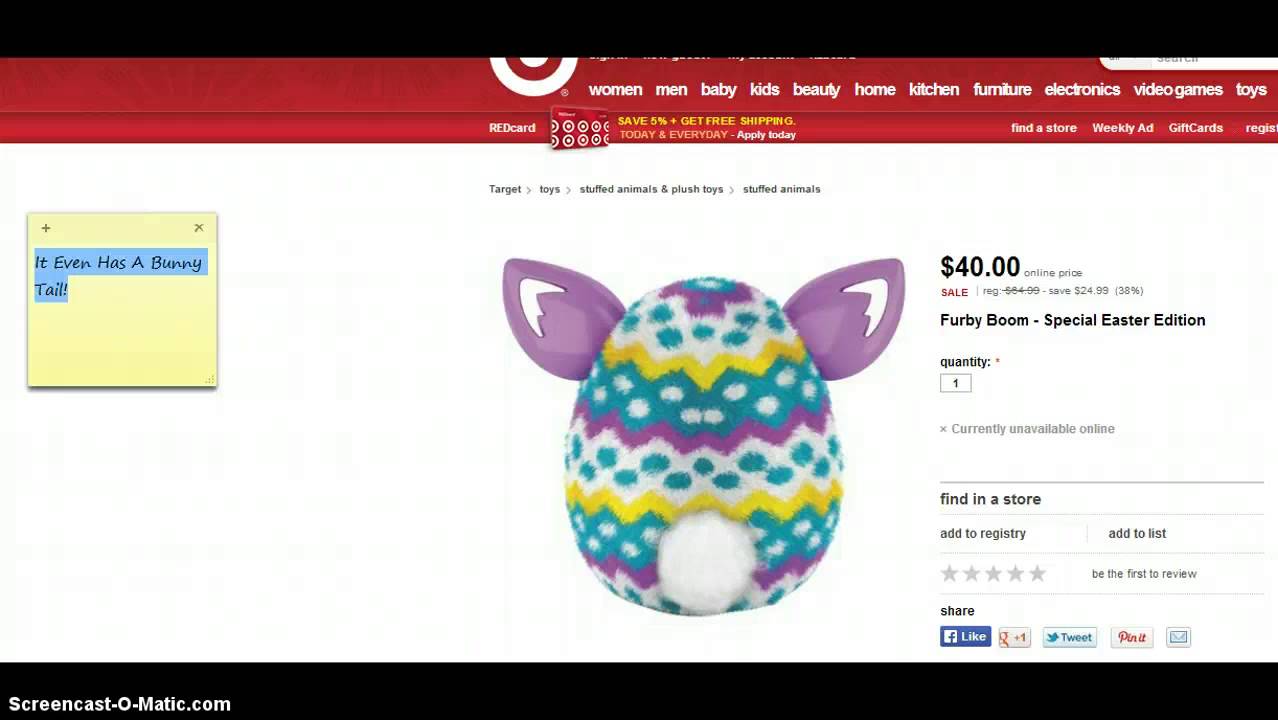The screenshot displays the interface of a retail website. The top and bottom of the screen are bordered by horizontal black rectangles. Directly below the top black border is a thicker horizontal red bar extending across the screen. Slightly left of center, two thick white circles intersect the red bar from the top.

Below this, aligned to the right and across the top of the screen, is a menu list in white text featuring categories such as Women, Men, Baby, Kids, Beauty, Home, Kitchen, Furniture, Electronics, Video Games, and Toys. A thin gray line separates this menu from the content below. Still within the red bar but underneath the gray line is a line of text that is too small to decipher.

The main content area of the screen is predominantly white. Centrally located is a section in black font, captioned with "Stuffed animals." To the left, there is a blue square inset with white text that reads, "It even has a bunny tail!" Inside this square is a multicolored bunny resembling an Easter egg. The bunny has a flat bottom and features two purple ears, a white patch towards the top, and horizontal stripes in yellow, white with green circles, purple, green with white circles, and yellow again. It is adorned with a round white cotton ball tail.

On the right side of the image, the price of the bunny is displayed clearly: $40.